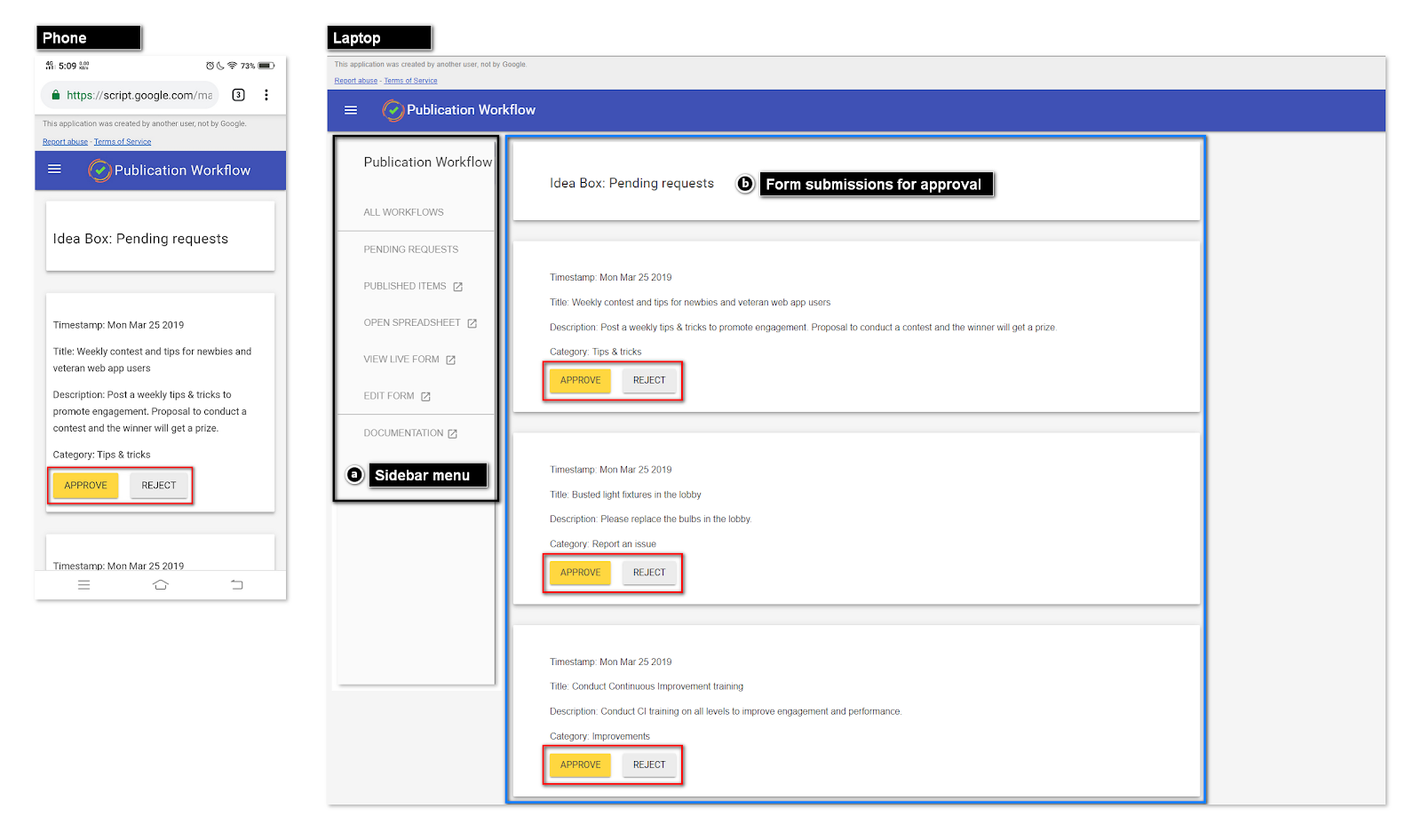The image showcases a webpage displayed on two different devices: a phone and a laptop.

**Phone Interface:**
- Location: Top left corner.
- Header: "Phone" written in white on a black background.
- URL: Displayed as "scripts.google.com."
- Notification: "This application was created by another user, not by Google," written in black text.
- Buttons: Two blue buttons labeled "Report Abuse" and "Terms of Service."
- Page Name: "Publication Workflow" written in white on a blue background with an icon that has orange, yellow, and a green tick.
- Content: "Idea Box Pending Request" written in black on a white background.
- Timestamp: "Monday, March 25, 2019."
- Title: "With Context and Tips for Newbies and Veteran Web App Users."
- Description: "Post a weekly tip and tricks to promote engagement. Proposal to conduct a contest and the winner will get a prize."
- Category: "Tips and Tricks."
- Action Buttons: 
  - "Approve" button in yellow.
  - "Reject" button in grey with a red outline.

**Laptop Interface:**
- Header: "Laptop" written at the top.
- Sidebar Menu: Located on the left side with a white background and black text outlined in a black square.
- Sidebar Options: "Publication Workflow," "All Workflows," "Pending Request," "Published Item," "Open Spreadsheet," "View Live Form," "Edit Form," "Documentation."
- Main Content:
  - Outline: Enclosed in a blue square.
  - Heading: "Idea Box Pending Request" written in black.
  - Label: "Form Submissions for Approval" with white text on a black background, labeled as "B."
  - Timestamp: "Monday, March 25, 2019."
  - Text: Matches the content from the phone interface.
  - Action Buttons:
    - "Approve" button in yellow.
    - "Reject" button in grey with a red outline.

The image effectively demonstrates the design consistency of the webpage across both mobile and desktop interfaces, highlighting key interactive elements such as the action buttons and workflow management features.